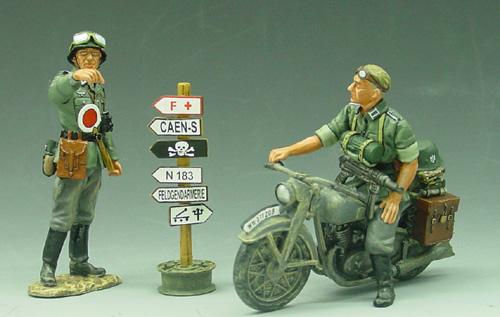This professionally photographed image showcases two intricately detailed army figurines from around the World War II era, one mounted on a gray and black motorcycle and the other standing on a platform designed to resemble the ground. The first figurine, possibly German due to the greenish-gray uniform, sports a helmet with goggles, an olive long-sleeve shirt and pants, knee-high black boots, and a brown pack slung over his shoulder. He points to the distance, with a white and red medallion symbolizing a medical badge on his chest. The second figurine, riding the motorcycle with rolled-up sleeves and blond hair, wears sunglasses pushed above his eyes and has a brown case attached to his bike, with a helmet resting behind him. Both figures appear to be part of a military clinic or medical unit.

Adjacent to the figures is a wooden signpost adorned with multiple directional signs: a red one with "F+" pointing left, black and white "CAEN-S" also to the left, a black sign with a skull and crossbones indicating danger, another white sign saying "N 183" pointing left, and several other indistinguishable indicators in various colors. The signs add a touch of narrative and situational context to the scene.